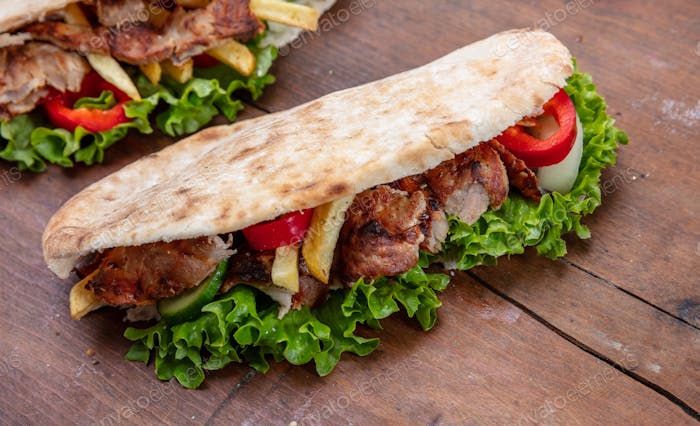The image showcases two mouthwatering pita sandwiches resting on a rustic, cracked wooden table. The primary sandwich, fully visible in the center, features a soft, beige flatbread with brown spots. The pita is generously filled with juicy grilled chicken, vibrant slices of red peppers, potentially some squash, crunchy cucumbers, and fresh green romaine lettuce. Added to the medley are crisp french fries, tangy white onions, and a hint of hard-boiled egg peeking from underneath the peppers. The secondary sandwich, positioned partially in the background, mirrors the ingredients of the first but is only partially visible, revealing its colorful filling against the aged, streaked wooden surface. The texture and color of the wooden table enhance the presentation of these delectable sandwiches, making them appear even more inviting.